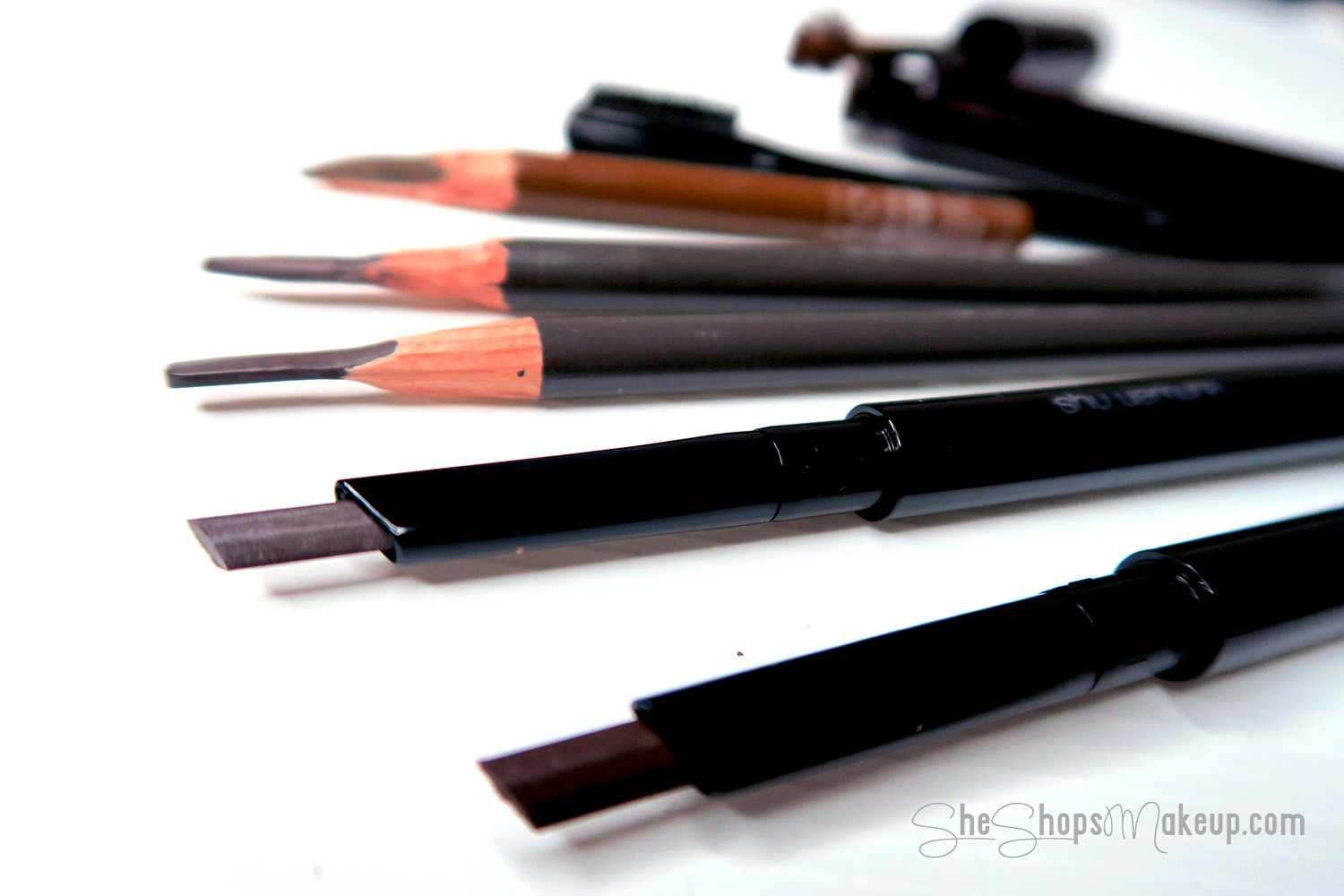The advertisement photograph features an array of makeup pencils, art pencils, and pens arranged in a fan formation originating from the right side and spreading across a pristine white surface. At the bottom right corner, the URL "SheShopsMakeup.com" is prominently displayed in gray letters, with the initials 'S' and 'M' stylized in cursive. In the foreground, there is a black pen-like contraption with a rectangular piece of lead sticking out, tilted downwards, followed by a similar device with a lighter gray lead. Behind these, there are two sharpened gray pencils with unusually long exposed leads, possibly for artistic use. Next up is a brown pencil with white text near its base and what seems to be brown ink. The entire collection, which includes a mix of black twist pens and another pen-like gadget, fans out beautifully, creating a dynamic and visually engaging composition.